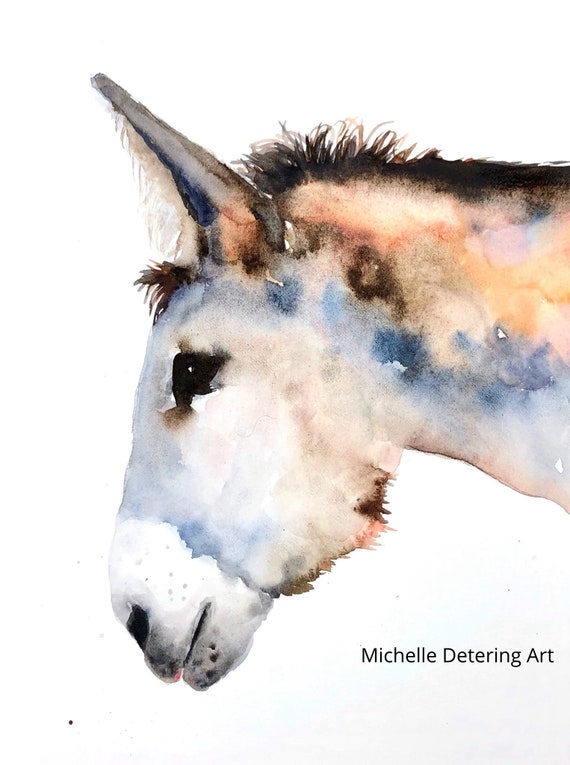This is an impressionistic watercolor painting of a donkey, signed "Michelle Deterring Art" in the bottom right corner. The background is predominantly white with occasional black and grey speckles. The donkey is depicted in left profile, showing only its neck, face, and part of its ears. Its head is angled downward toward the bottom left of the frame. 

The donkey's fur is a vibrant mix of blue, brown, white, and orange with occasional hints of pink and yellow. It has a distinct blue highlight around the center of the neck and near the face. The ear is pointed and tilted slightly forward, featuring a dark blue highlight and white tufts of fur poking out. The short mane on top of its head exhibits black hairs, resembling a mohawk, and black expressive eyes sit above a white and grey-speckled snout, ending in a black nose.

The muzzle appears whiter with subtle grey contours, and brown and pink tufts of fur adorn the chin area. The painting showcases the animal's textured fur, both in its mane and around its ears, making it almost a realistic rendition despite its impressionistic style. The overall effect of the watercolor technique gives the donkey a soft, marbled appearance, blending the vibrant colors smoothly across its form.